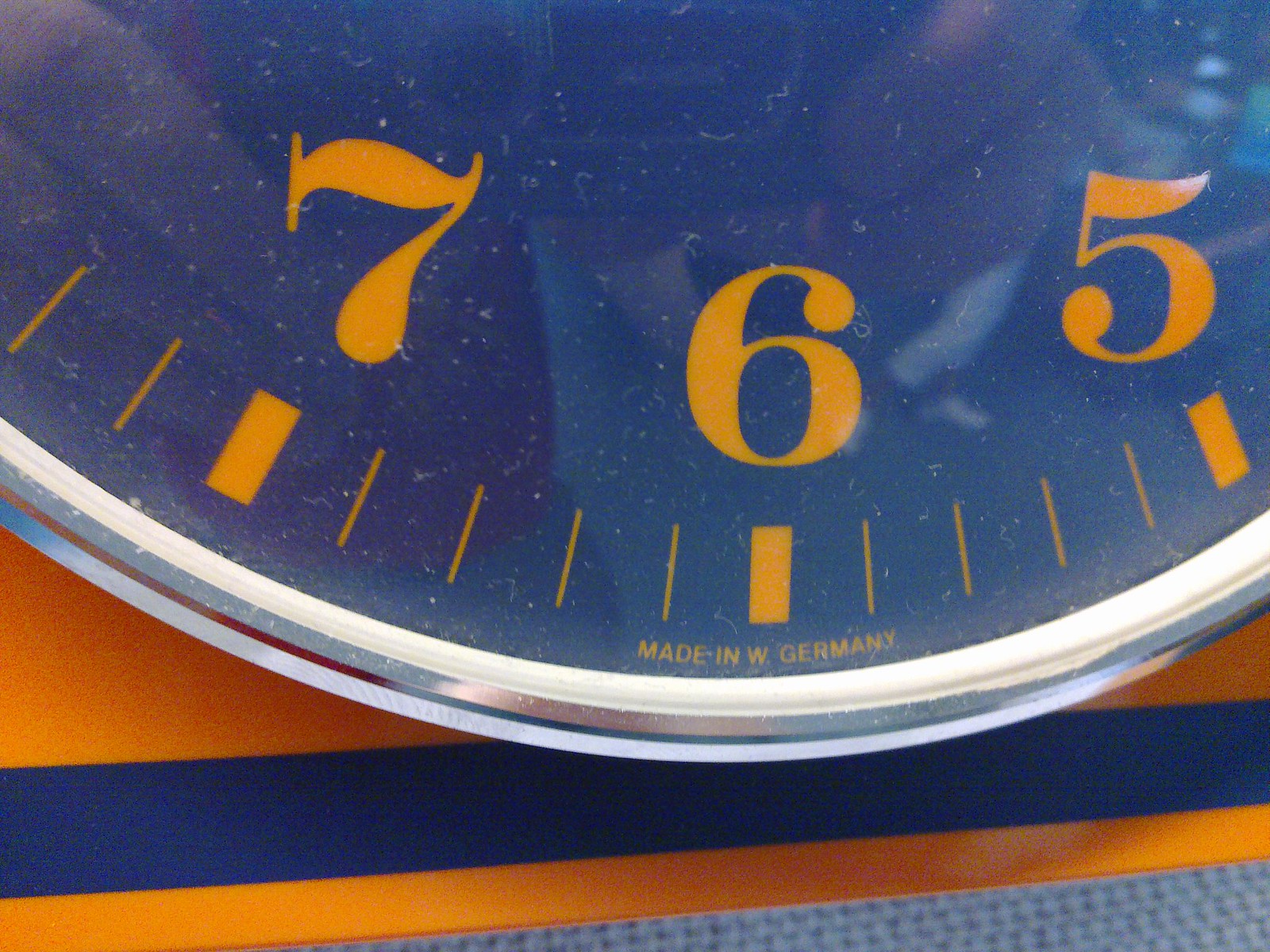A close-up image showcases the intricate details of a clock's bottom portion. The clock's face, rendered in a striking blue, is adorned with elegant golden numbers that gleam in the light. A tiny inscription at the bottom reads "Made in West Germany," hinting at the clock's origin and potentially its vintage. Encasing the blue clock face is a luxurious gold chrome rim, which is bordered by a pristine white outer edge, providing a stark yet complementary contrast. The clock rests on a fabric with a pattern of yellow and blue stripes, below which a whitish cloth weave adds a subtle texture to the background, enhancing the overall aesthetic of the composition.